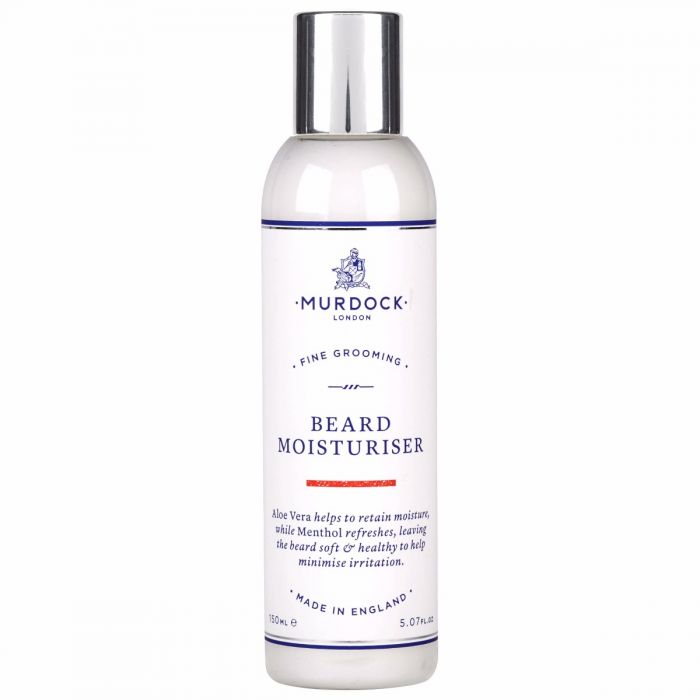This image is a detailed photograph of a grooming beauty product, specifically a beard moisturizer. The product is housed in a tall, slender white bottle with a polished silver cap. A substantial label wraps around the bottle, predominantly featuring a design motif of a man seated, etched above the name "Murdoch London Fine Grooming" in blue print. The central label prominently marks the product as a "Beard Moisturizer," followed by descriptive text in blue, separated by a striking reddish-orange band. The text highlights that aloe vera helps retain moisture, while menthol refreshes, consequently leaving the beard soft and healthy, and minimizing irritation. The label also notes that the product is made in England and lists the volume as 150 milliliters or 5.07 fluid ounces. The entire image is set against a completely plain white background, providing no additional context or setting.